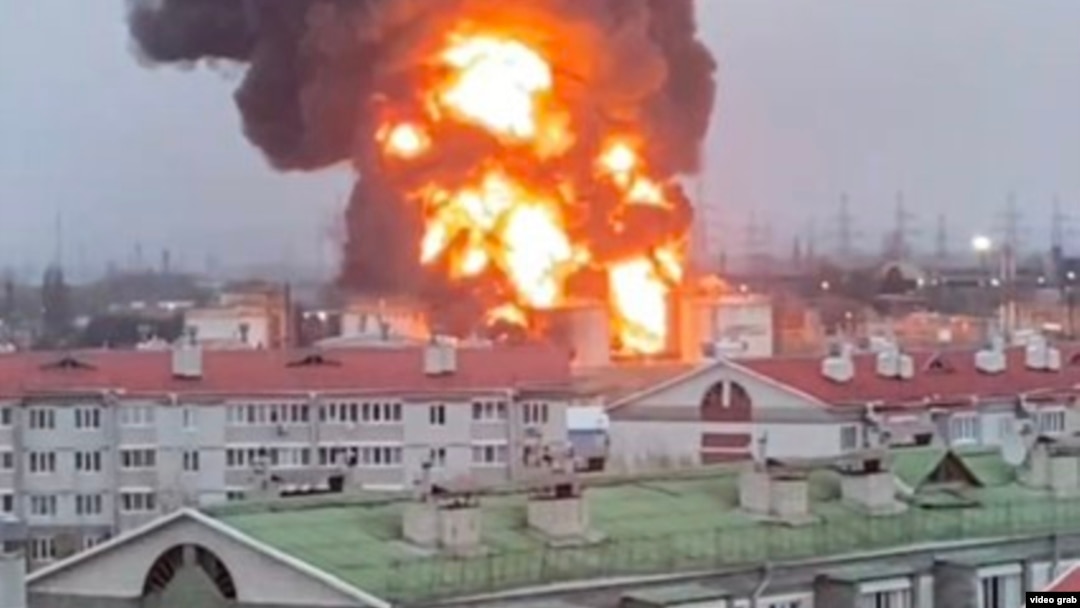A massive explosion engulfs a residential area, with towering flames and a thick black cloud of smoke rising dramatically against a gray, overcast sky. The foreground features two prominent buildings—one with a red roof, the other with a green one—amongst an array of apartment complexes with similarly red-roofed structures. In the background, a network of power lines is visible, adding to the chaotic scene. The image captures the tragic scale of the fire, likely causing significant impact to the lives of residents in the area. A small text in the bottom right-hand corner reads "video grab," hinting at the source of the image. The devastation evoked by this scene raises poignant questions about the cause and aftermath of the explosion.